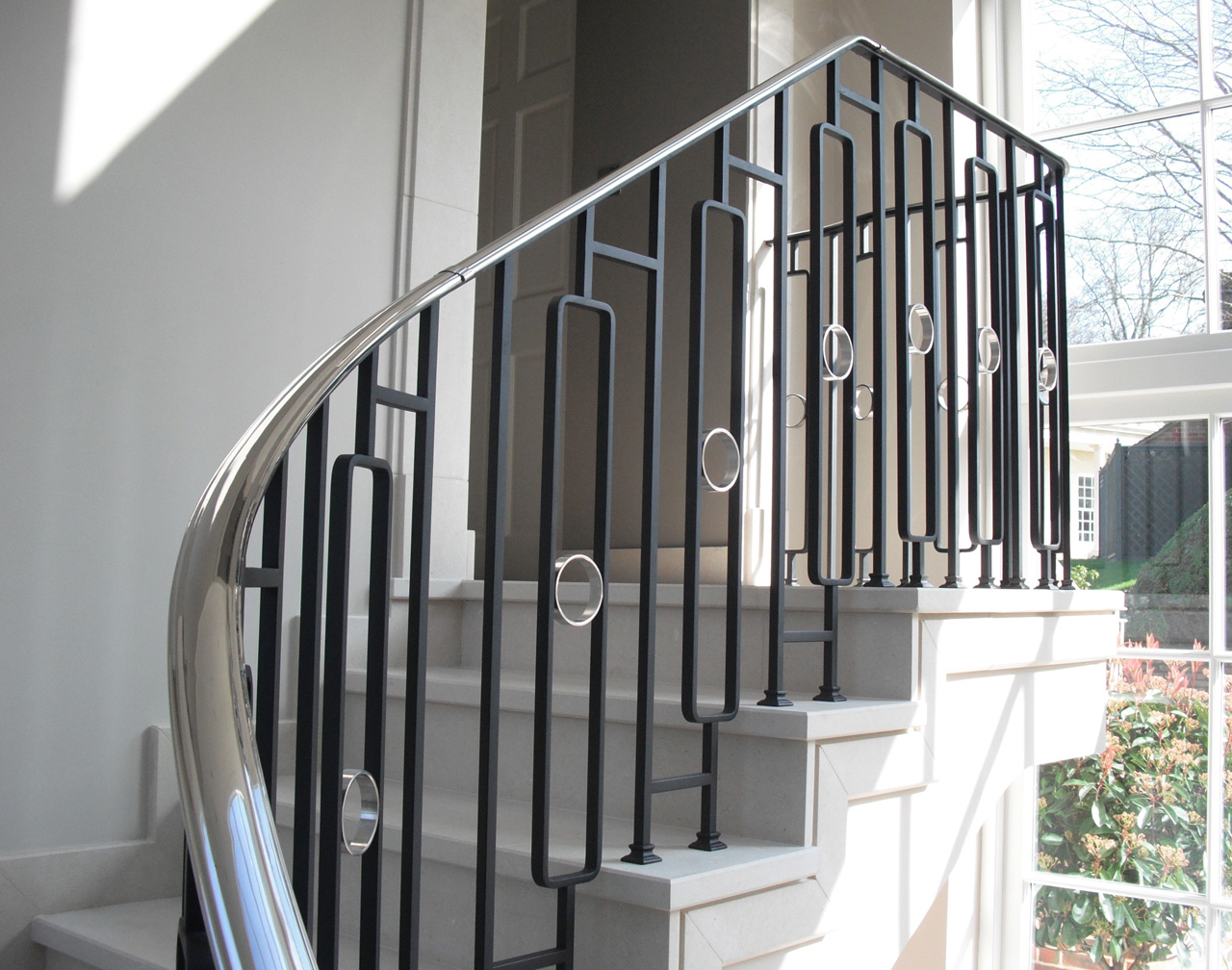This image captures a well-lit interior staircase, potentially inside a home's atrium or entrance hall. The focal point is a winding staircase with polished white marble steps leading to a darkened doorway on an upper floor. The staircase features a distinctive handrail composed of dark wrought iron balusters interspersed with chrome rings and topped with a sleek silver handrail. On the right side of the image, a large pane-glass window extends from the floor to the ceiling, allowing abundant sunlight to stream in and offering a view of a garden below. This garden area showcases green bushes, orange flowers, and is enclosed by a brown fence with barren trees visible beyond. The left wall of the interior is white with a streak of light due to the bright outdoor scenery shining in through the window. Overall, this photograph strikingly highlights the elegant staircase and its intricate handrail design against the natural beauty of the garden seen through the adjacent window.